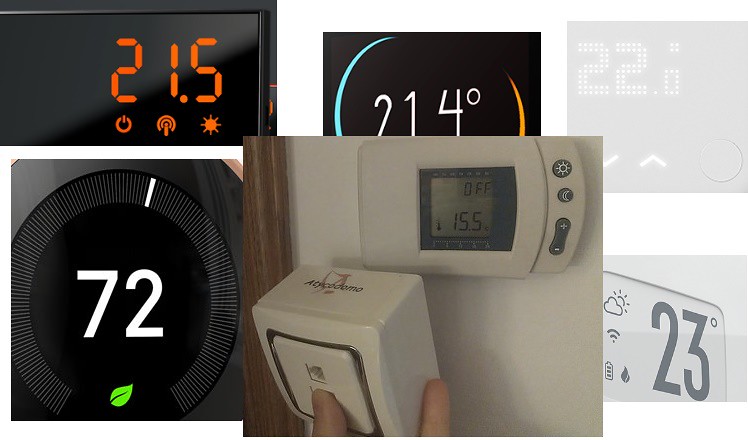The image showcases six distinct digital thermostat faces, each varying in design and color. Among them, one is identified as a Google Nest thermostat, recognized by its sleek and modern interface. Another features a classic digital face reminiscent of older digital models. The remaining four thermostats are similar in design, likely smart thermostats, yet each one is differentiated by unique color accents. The thermostats are arranged evenly, occupying equal space within the image. Each device prominently displays temperature readings, with some showing temperatures to the nearest decimal point while others round to the nearest whole degree. The focus of the image is on the digital displays, highlighting the precision and varied presentation of temperature information across different thermostat models.